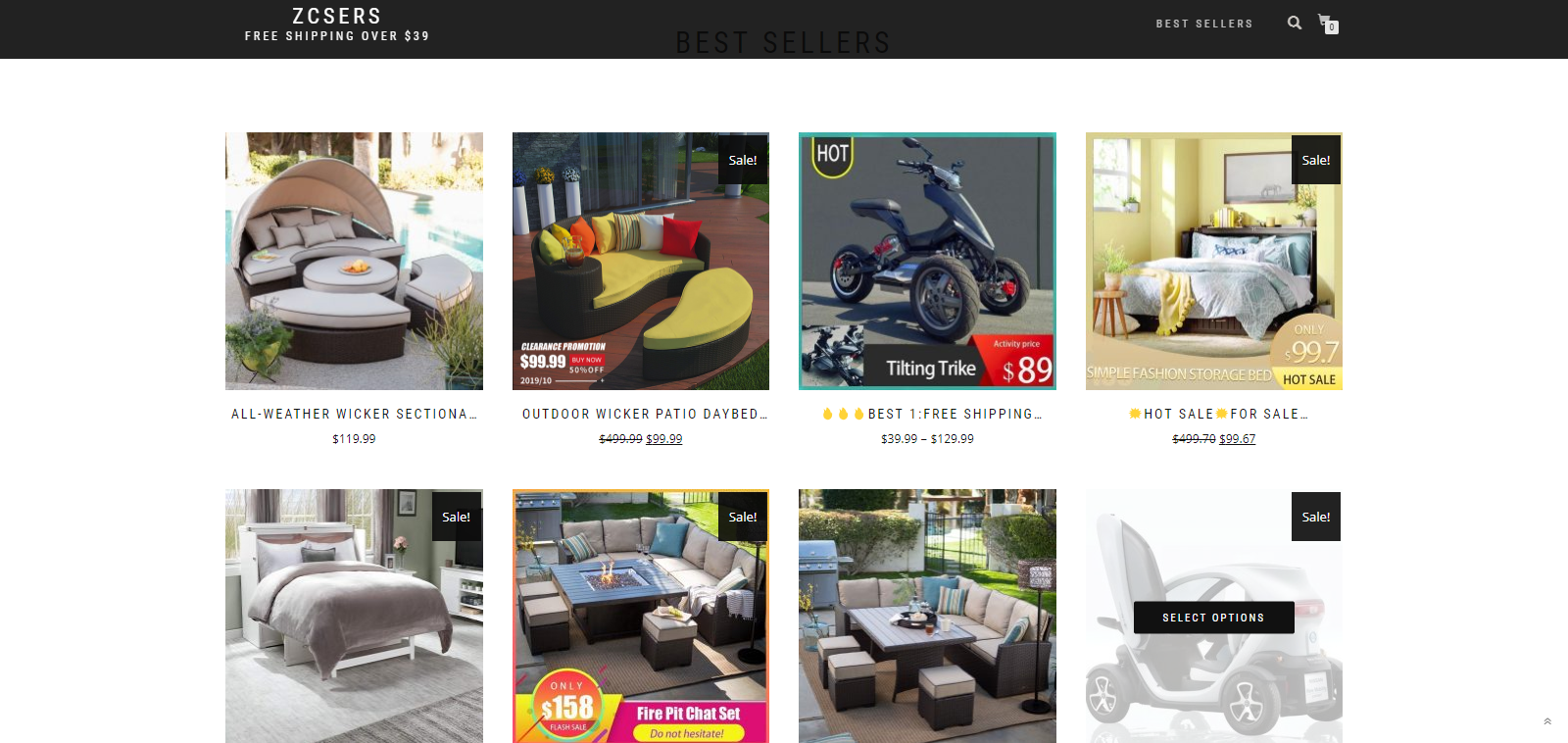This is a detailed webpage screenshot from the SCSERS website. At the top left corner of the main banner, the site logo 'SCSERS' is prominently displayed. Directly below this, a promotional banner announces "Free Shipping Over $39". On the right-hand side of the top banner, there are three interactive elements: a shopping cart icon, a search button, and a link to the 'Best Sellers' section.

In the center of the page, there are eight distinct boxes showcasing items for sale on the website. Each box features a different product. The top row includes:

1. An all-weather wicker recreational outdoor set priced at $118.99. The text appears small and hard to read but seems to be accurate.
2. An outdoor wicker patio daybed, highlighted with "Best One" and indicating it includes free shipping. Interestingly, this product image includes a child’s tricycle.
3. A bedroom set, with a clear visual representation emphasizing its design and composition.

On the lower row, from left to right, the products displayed are:
1. Another stylish bedroom set, offering a different aesthetic compared to the one above.
2. An outdoor patio set priced at $158.00.
3. Another outdoor patio set with distinctive features suitable for different preferences.
4. A small electric car, resembling a tiny golf cart, perfect for fun rides or easy commutes around a private estate.

Each image is designed to catch the eye and provide a preview of the diverse range of products available on the SCSERS website.